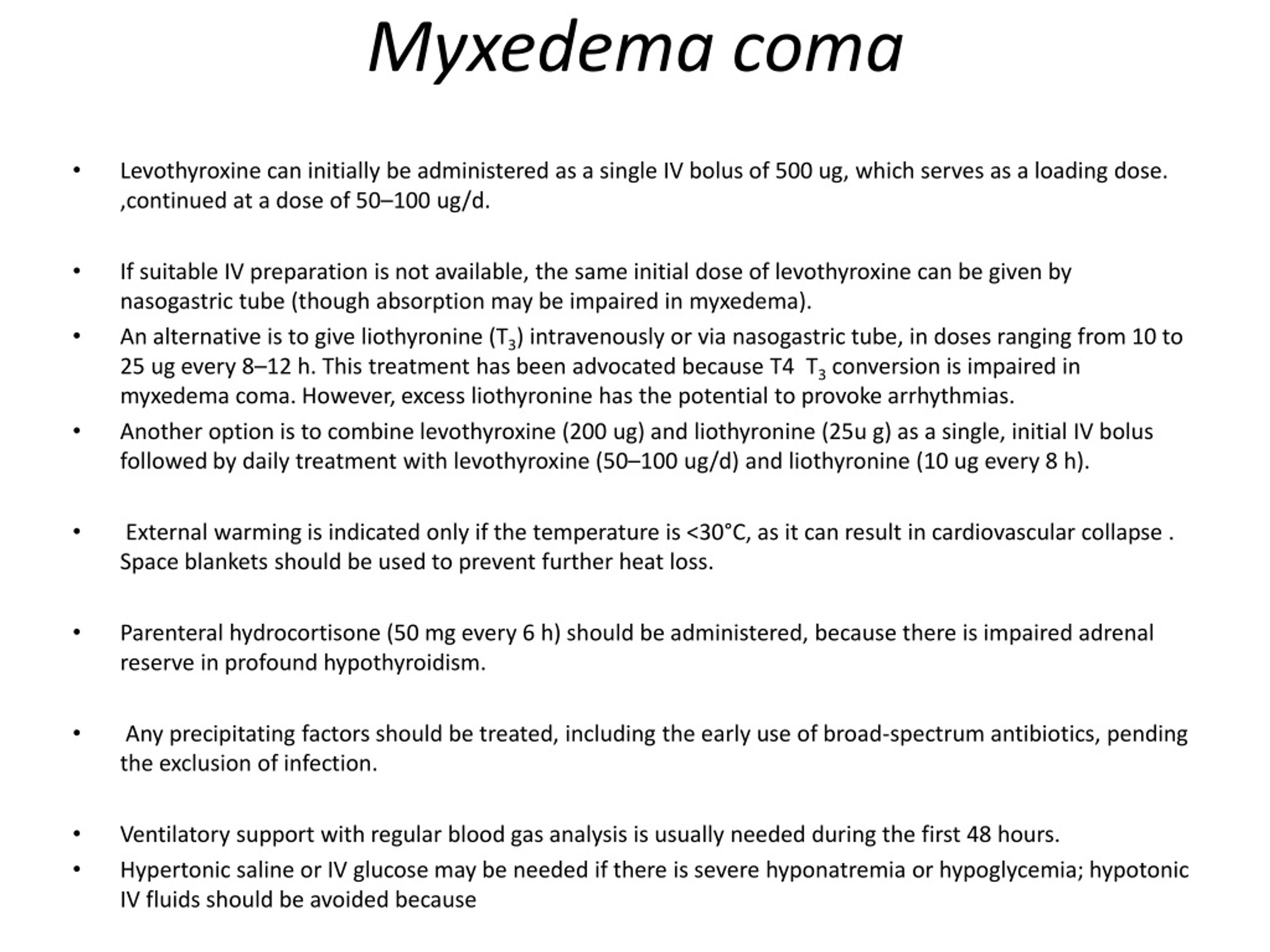This is a detailed screenshot consisting of text only, likely taken from a medical document or presentation about the treatment of Myxedema. At the very top and centered in large, italicized font is the heading "Myxedema."

On the left side, there are approximately 9 or 10 bullet points summarizing treatment options:

1. **Levothyroxine Administration:** Initially, Levothyroxine can be administered as a single IV bolus of 500 micrograms (UG), which serves as a loading dose. This is then followed by a continued dose of 50 to 100 micrograms per day (UGD).

2. **Alternative Administration via Nasogastric Tube:** If IV preparation is unavailable, the same initial dose of Levothyroxine can be given via a nasogastric tube. However, it is noted that absorption may be impaired by Myxedema.

3. **Liothyronine (T3) Alternative:** An alternative treatment is to administer Liothyronine (T3) either intravenously or through a nasogastric tube in doses ranging from 10 to 25 micrograms every 8 to 12 hours. This treatment is recommended because T4 to T3 conversion is impaired in Myxedema coma. However, it is cautioned that excess Liothyronine has the potential to provoke arrhythmias.

The remaining bullet points, though not detailed here, continue to outline medical protocols aimed at managing and treating patients experiencing a Myxedema coma.